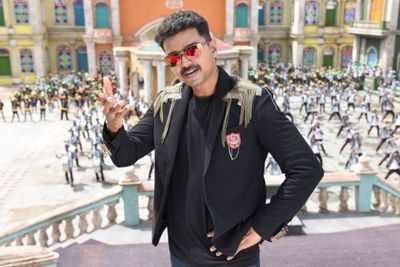A man of seemingly Indian descent stands confidently on the landing of a grand double stairwell, which splits left and right, reminiscent of palace architecture. The sun shines brightly, illuminating his striking appearance. He dons a black jacket adorned with fringe or tassels on the shoulders, resembling the shoulder coverings of a general. Attached to his left pocket is a rose, adding a touch of elegance. His beige-ish skin contrasts with his black curly hair and his reflective reddish-orange sunglasses. His right hand is pointed outward in a gesticulating pose, while his left hand rests on his hip. Underneath the jacket, he wears a black t-shirt and black pants, completing his ensemble. Behind him lies a bustling courtyard or plaza, possibly in Italy, where brightly colored buildings frame the scene. Groups of people are engaging in coordinated activities, such as dancing and exercising, hinting at a choreographed performance, possibly for a Bollywood movie. Despite the lively backdrop, the man looks directly at the camera with a serious expression, creating a captivating focal point amid the vibrant surroundings.